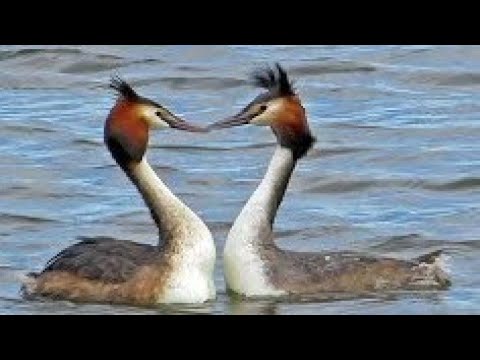This striking photograph captures two birds, appearing almost as mirror images of each other, as they gracefully float on a serene body of water. The exact type of water—whether a river or the ocean—remains unclear, adding an element of mystery to the scene. The birds are elegantly poised, each with a long, white neck reminiscent of a goose's, arched gracefully in a swan-like manner.

One bird's plumage is predominantly brown with a touch of white on its neck, while the other showcases black feathers that contrast beautifully with its white neck. Both birds feature a distinctive reddish hue on their heads, crowned with black feathers that stand upright like a cowlick. The birds are positioned in such a way that their beaks are almost touching, creating a harmonious and symmetrical composition. Their serene presence on the water and their unique coloring make them a captivating sight to behold.